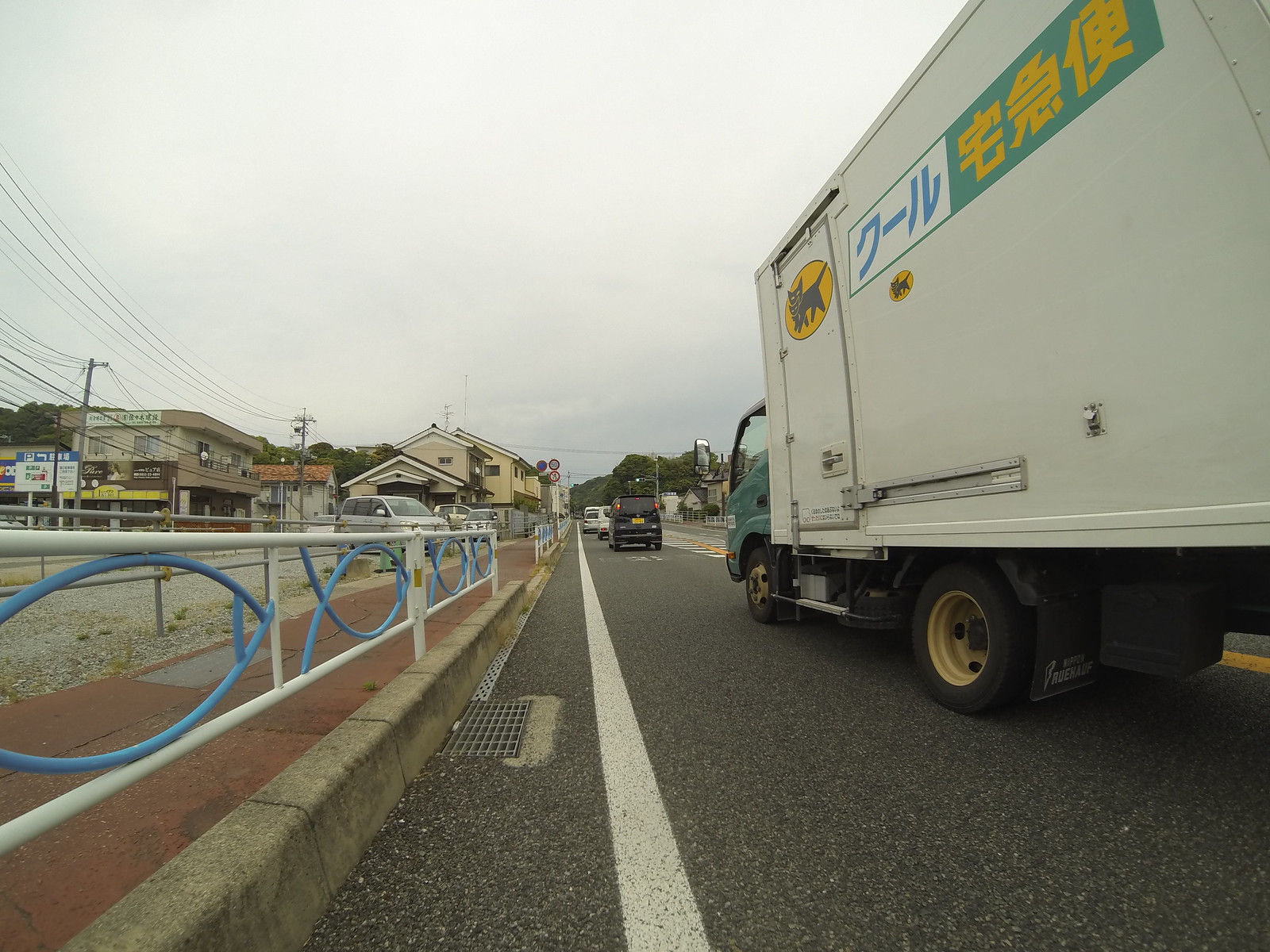This photograph, taken in Japan, showcases a street scene with a sidewalk prominently running through the middle of the frame. The sidewalk is defined by red brick or stone paving, bordered on the left by a row of homes and parked cars. On the right side of the image, the street itself hosts various vehicles, including a notable Japanese semi-truck featuring a cat logo. Further down the road, more cars can be seen receding into the horizon. Adding to the urban context, a storm drain grate is visible at the curb. The scene is enveloped in a gray, overcast atmosphere, contributing to the subdued mood of the photograph.